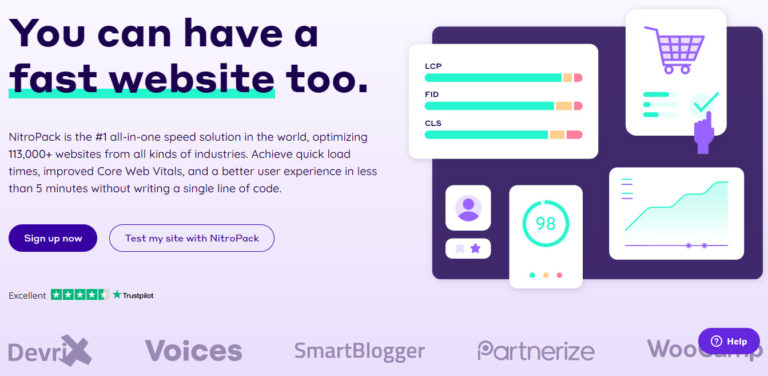The top section of the image features a light purple background with bold black text in large letters that reads: "You can have a fast website too." The phrase "fast website" is underlined in teal. Below this, the text states: "Nitro Pack is the number one all-in-one speed solution in the world, optimizing 115,000 websites from all kinds of industries. Achieve quick load times, improve Core Web Vitals, and enjoy a better user experience in less than five minutes without writing a single line of code."

Beneath this description, there is a prominent blue button labeled "Sign Up Now". Next to it, a purple rectangle button states "Test My Site with Nitro Pack". Below these buttons, the text reads: "Four out of five stars – Excellent."

On the right side of the image, there is a dark purple square containing a white box with a shopping cart icon inside. Beneath the shopping cart, there is a teal checkmark alongside a hand with a light purple finger pointing towards it. 

Underneath this, there is a white box featuring a teal graph with a purple line at the bottom, indicating performance metrics.

Finally, a purple button at the bottom of the image reads "Help".